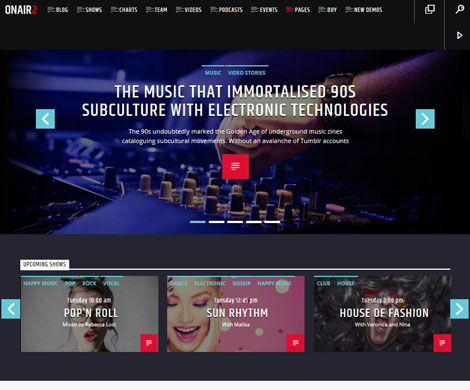Caption: 

A promotional pop-up screen for a music performance event, featuring a black background with the title, "The Music that Immortalized 90s Subculture with Electronic Technologies." Dominating the screen is a photo of an auditorium filled with numerous empty seats, hinting at the anticipation of an upcoming event. Below the main image are three smaller boxes, each displaying unique music genres or performance names: "Pop and Roll," "Sun Rhythm," and "House of Fashions." This visually intriguing advertisement seamlessly blends nostalgia with modern electronic music, beckoning viewers to explore a rich tapestry of 90s-inspired performances.